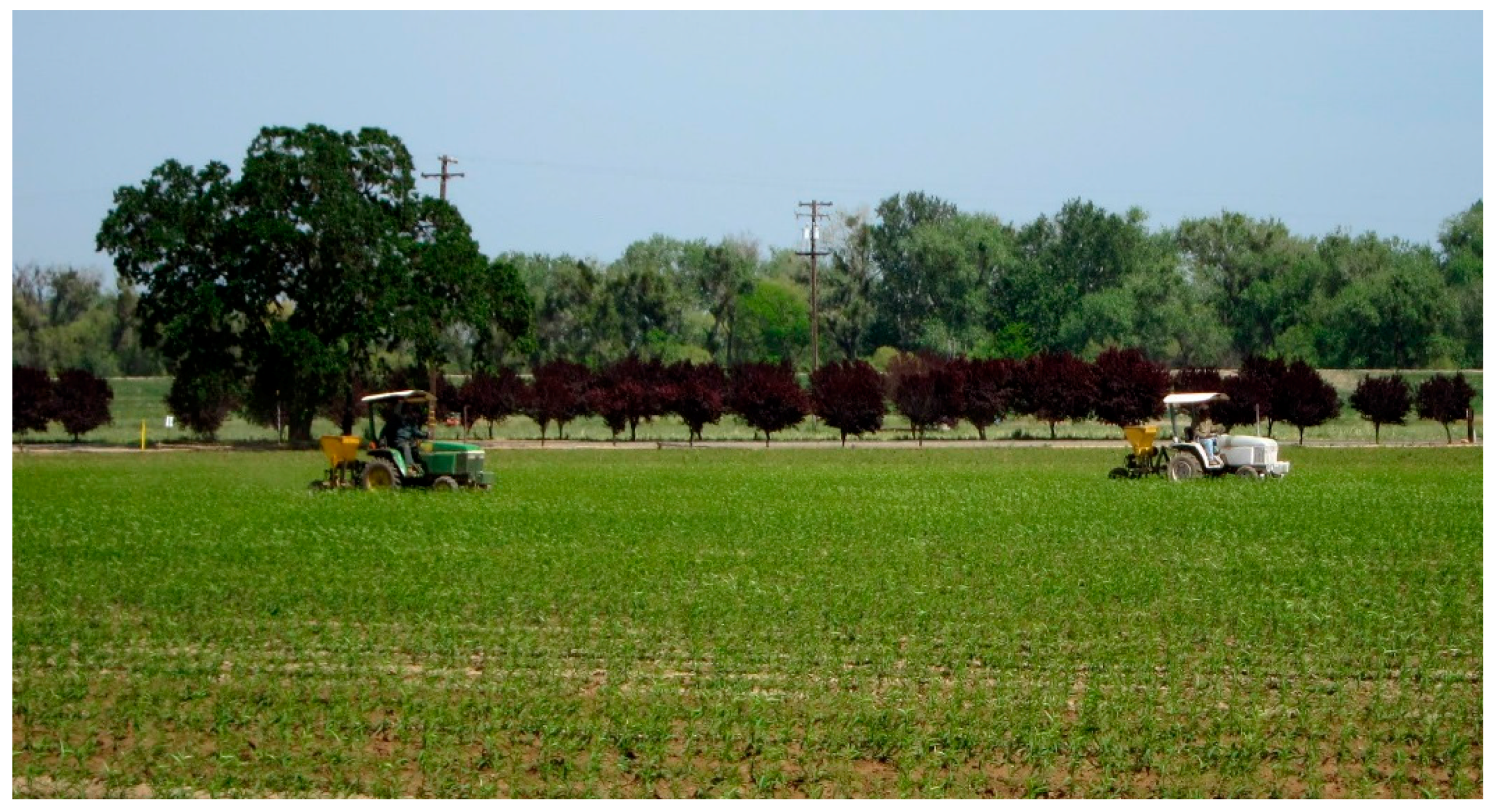In this sunlit, peaceful farmland scene, two tractors are diligently tending to a green field. The image is wider than it is tall, capturing a panoramic view of the agricultural activity. On the right side, there is a white four-wheel tractor with a protective cover to shield the driver from the sun. It's equipped with a yellow attachment that resembles a seeder, indicating it might be planting crops. Further to the left, several rows away, a second tractor, typically John Deere green with yellow accents, mirrors the first tractor's activity under its own shade cover.

The field itself is lush with young plants that are visibly above the soil, showcasing early growth stages. In the distant background, a line of reddish-burgundy trees, possibly flowering plums, marks the boundary of the property, and behind them, towering green deciduous trees stand tall. Power lines and poles cut across the field, suggesting an intersection nearby, and a yellow post is visible to the left of the green tractor. The bright blue sky overhead is clear of clouds, emphasizing the serene and sunny atmosphere of this agricultural landscape.